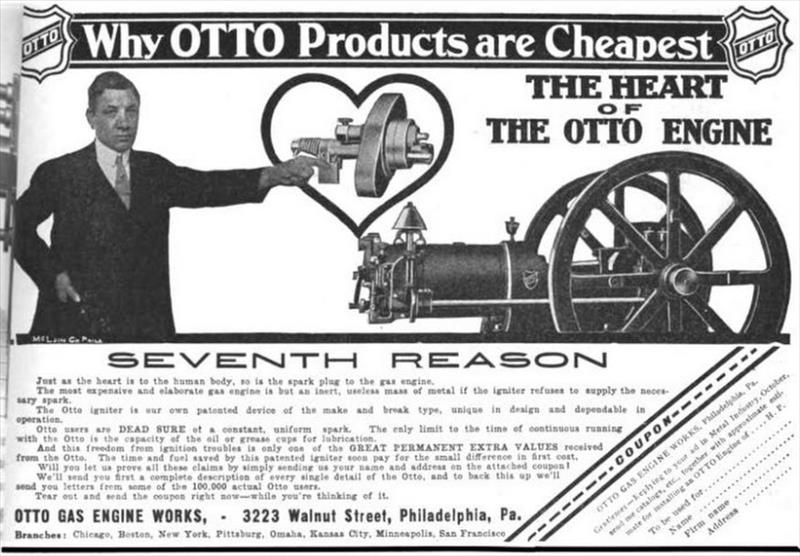This black-and-white vintage advertisement, possibly from an old magazine, showcases "Why Auto Products Are the Cheapest" with emphasis on "Auto" displayed within a shield-like logo at the top left and right corners. A well-dressed man, in a suit with a white collared shirt and tie, stands prominently in the center. He has short, combed-over hair and appears Caucasian. With his right hand in his pocket, he uses his left hand to point toward a detailed illustration of a dark-colored metal auto engine, described as "The Heart of the Auto Engine." The engine is adorned with gears resembling wooden wheels and intricate components, suggesting it is wheeled around. Below this illustration, it states "7th Reason" in black text and provides the address: Auto Gas Engine Works, 3223 Walnut Street, Philadelphia, PA. Despite some text being too small or blurry to read, the style and layout of this ad give it a retro 1960s feel with classic monochromatic design and detailed engineering sketches.